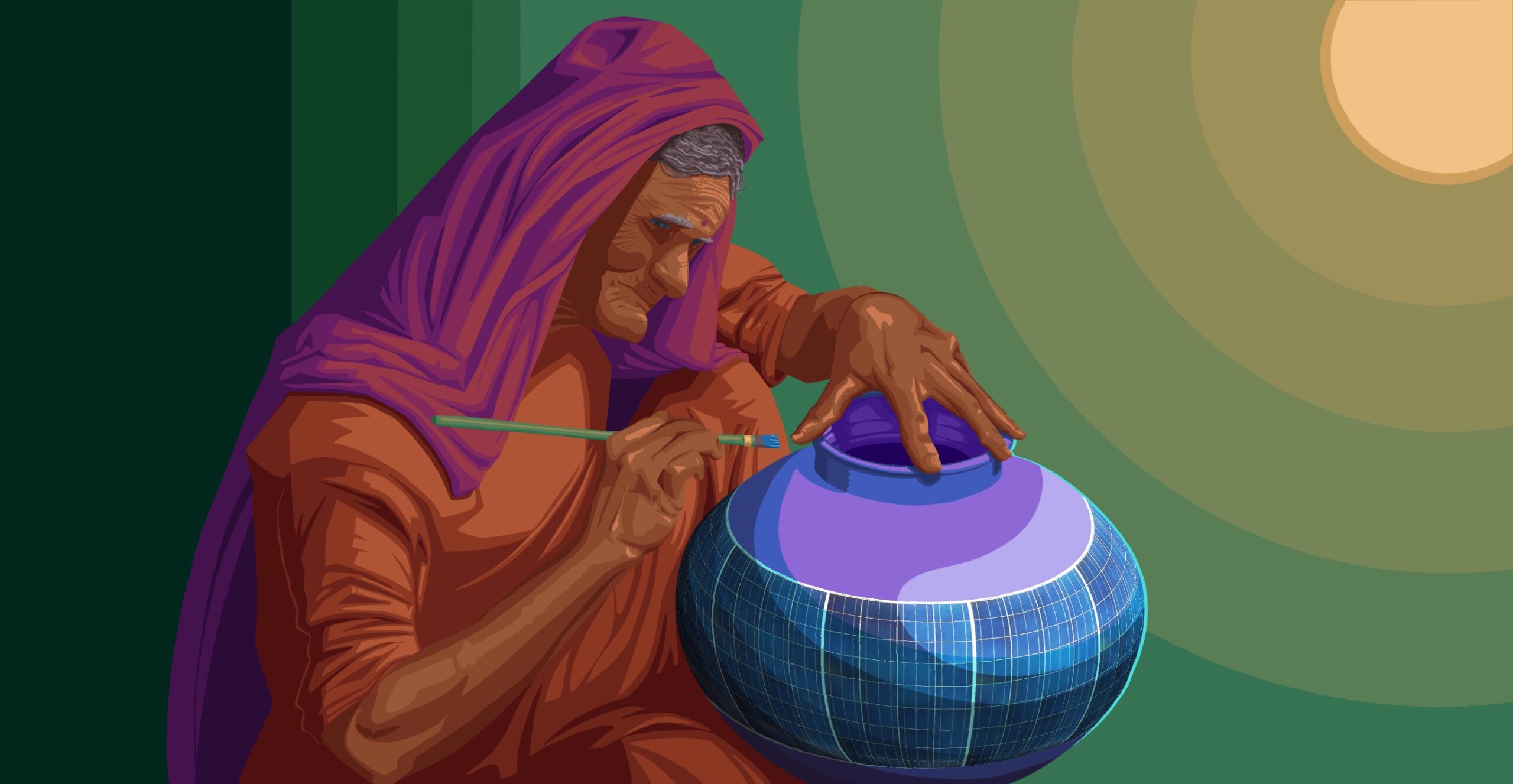In this digital illustration, an elderly Indian woman with a wizened, dark brown complexion and prominent facial features is meticulously painting a large, ornate vase. Her gray hair frames her face, partially concealed by a dark purple headscarf with reddish highlights, which trails down past her waist. The woman is dressed in a medium-tone orange gown, and her right hand delicately holds a green paintbrush tipped with blue paint. Her left hand steadies the vase resting in her lap, which features a large purple rim and a white and blue crisscross pattern. The background is a gradient starting with a golden circular halo in the upper right corner, transitioning through light green to dark green towards the left, giving the impression of a radiant, round sun.